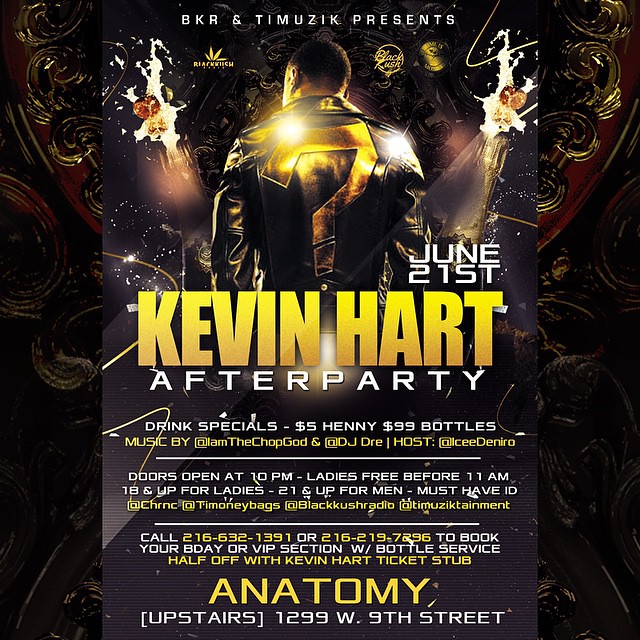This detailed flyer for a Kevin Hart after-party features a large, dark-themed image with black and brown tones. At the top, small white text reads "BKR and Timusic presents." Below this, the image shows Kevin Hart from behind, sporting short black hair and a black leather jacket adorned with a glowing gold and brown question mark. The backdrop includes champagne bottles popping and lens flares for added effect.

In the middle of the flyer, text indicates the event date, "June 21st," followed by "Kevin Hart" in large yellow block letters. Just below, in white all-caps, it reads "AFTER PARTY." Additional details include a list of drink specials like "$5.00 Henny" and "$99 Bottles," along with music by "@I'mTheChopGod" and "@DJDre," hosted by "IC D-Low."

Further down, information about door openings and admissions is provided: "DOORS OPEN at 10 p.m. LADIES FREE before 11 p.m., 18 and up for ladies, 21 and up for men, must have ID." For reservations, it lists the phone numbers "216-632-1391" and "216-219-7296" to book a B-Day or VIP section with bottle service, mentioning "Half off with Kevin Hart ticket stub." The flyer concludes with the name of the club, "ANATOMY," in large yellow letters, and the address "UPSTAIRS, 1299 West 9th Street," at the bottom.